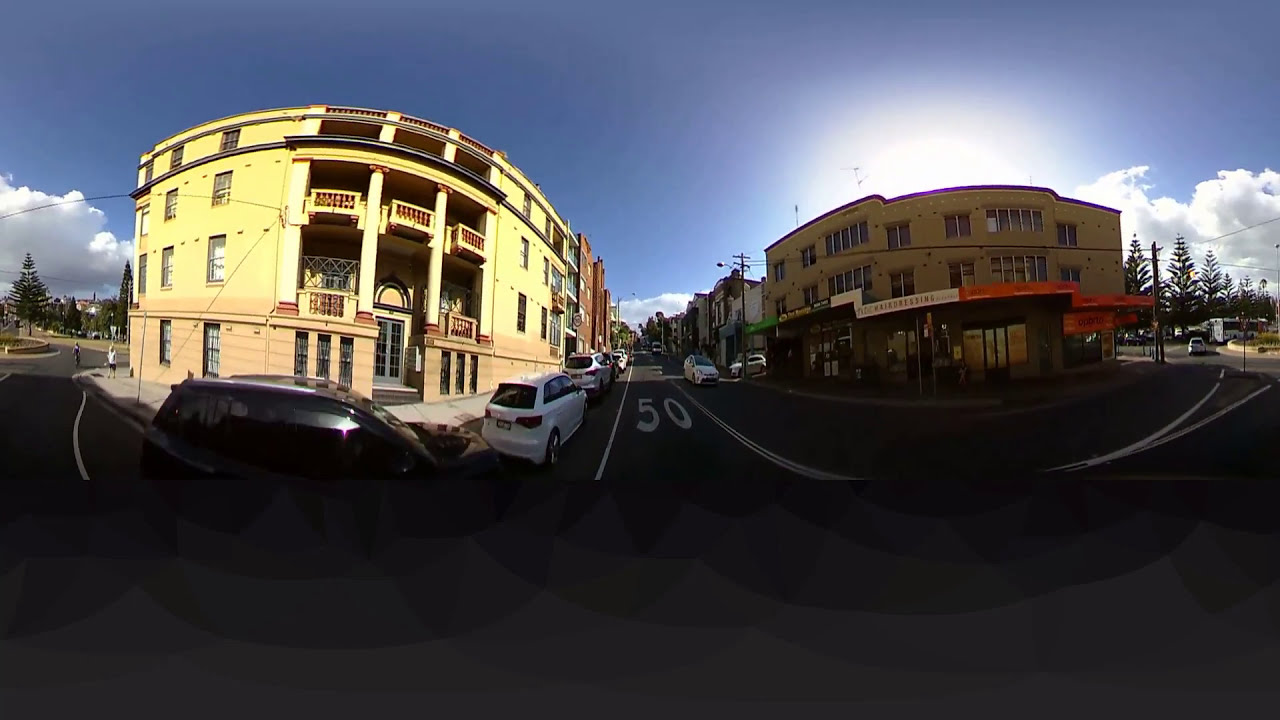This 360-degree panoramic image captures a vibrant urban street scene, viewed from possibly the dash of a motorcycle or car, with a distinct fisheye lens effect that distorts the surrounding buildings into a wavy, rounded appearance. The street, marked with white lines and the number "50" on either side, is a black-gray color and suggests a speed limit, possibly in kilometers per hour, indicating the location may not be American. Flanking the street are a series of older buildings, likely in a South American or Spanish style, characterized by their yellowish hues and well-kept facades.

To the left, there's a distinctive three-story building that is bright yellow on the top two levels and orangish-brown on the bottom, featuring small balconies. This building could be residential, possibly apartments. On the right side, similar in height and style, are buildings with red, white, and other colorful awnings and banners, hinting at commercial spaces such as shops or restaurants beneath the apartments above.

The extreme fisheye view enhances the charming, interconnected nature of these urban structures. A few conifer trees frame the scene, and the sky above is a bright blue with scattered clouds near the horizon. The sun shines brightly, partially obscured by one of the buildings on the right, casting a pleasant glow over this quaint street. The overall setting suggests a bustling, yet well-preserved urban area, rich with character and possibly historical significance.